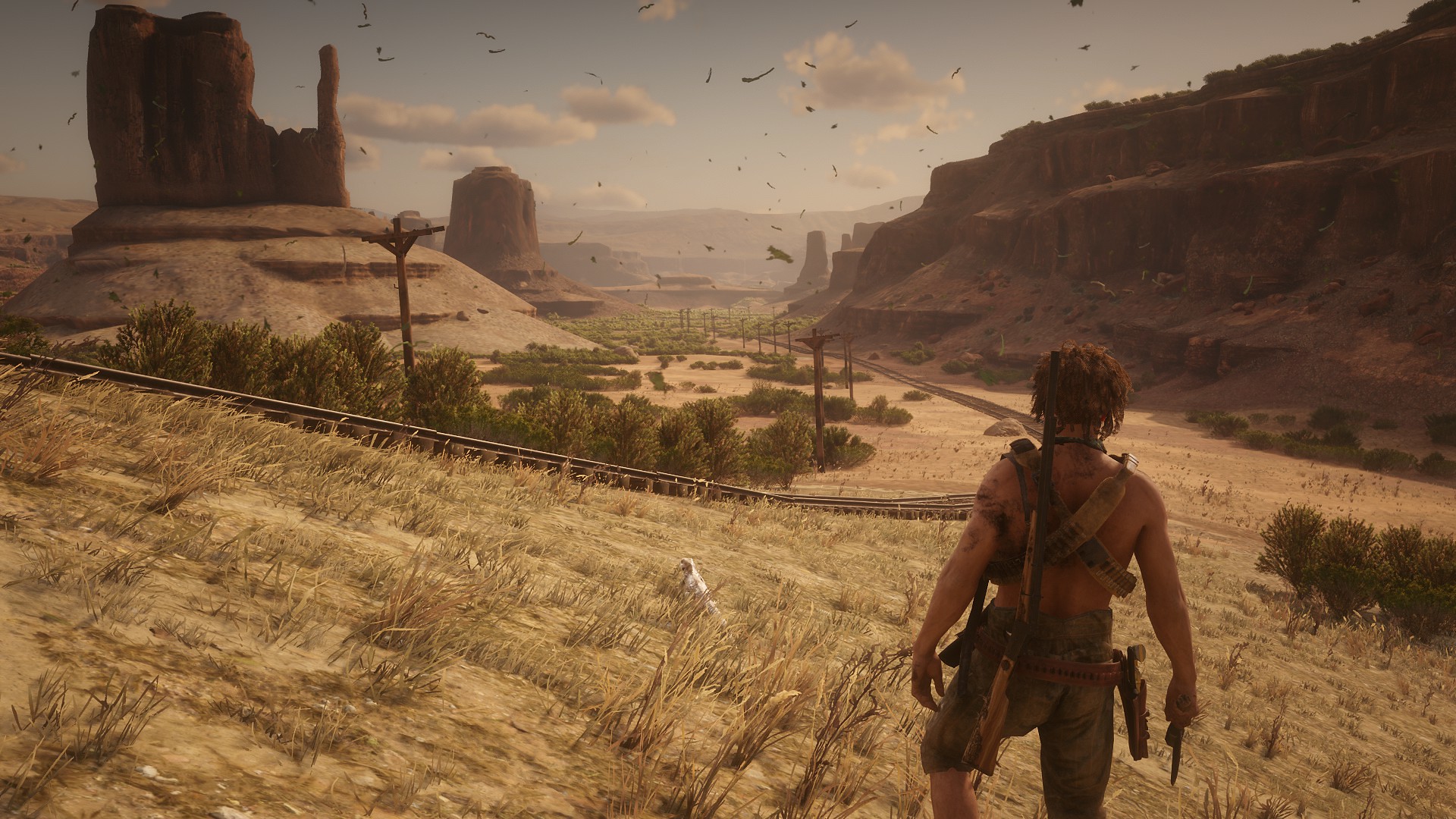The image appears to be a scene from a video game, showcasing a rugged, arid landscape. In the bottom right-hand corner stands the protagonist, a shirtless white male with brown scraggly or possibly ruddy hair. He is clad in tan, knee-high shorts and wears a leather harness for carrying weapons. In his right hand, he firmly grips a pistol, while a knife sheath is strapped to his waist. A rifle rests on his back. The character is facing away from us, surveying the expansive terrain laid out before him.

The environment features a mixture of dry, brown grass and sparse green vegetation typical of a desert or semi-arid region, reminiscent of California's landscape. Several distinctive geological features punctuate the scene, including a towering butte and a flattened mountain on the right. An abandoned set of train tracks runs through the middle of the image, hinting at a past era of industry. Remnants of old power lines, now devoid of cables, rise sporadically from the ground. The sky above is a clear blue with scattered white clouds, and multiple birds can be seen flying, adding to the scene's sense of desolate beauty.